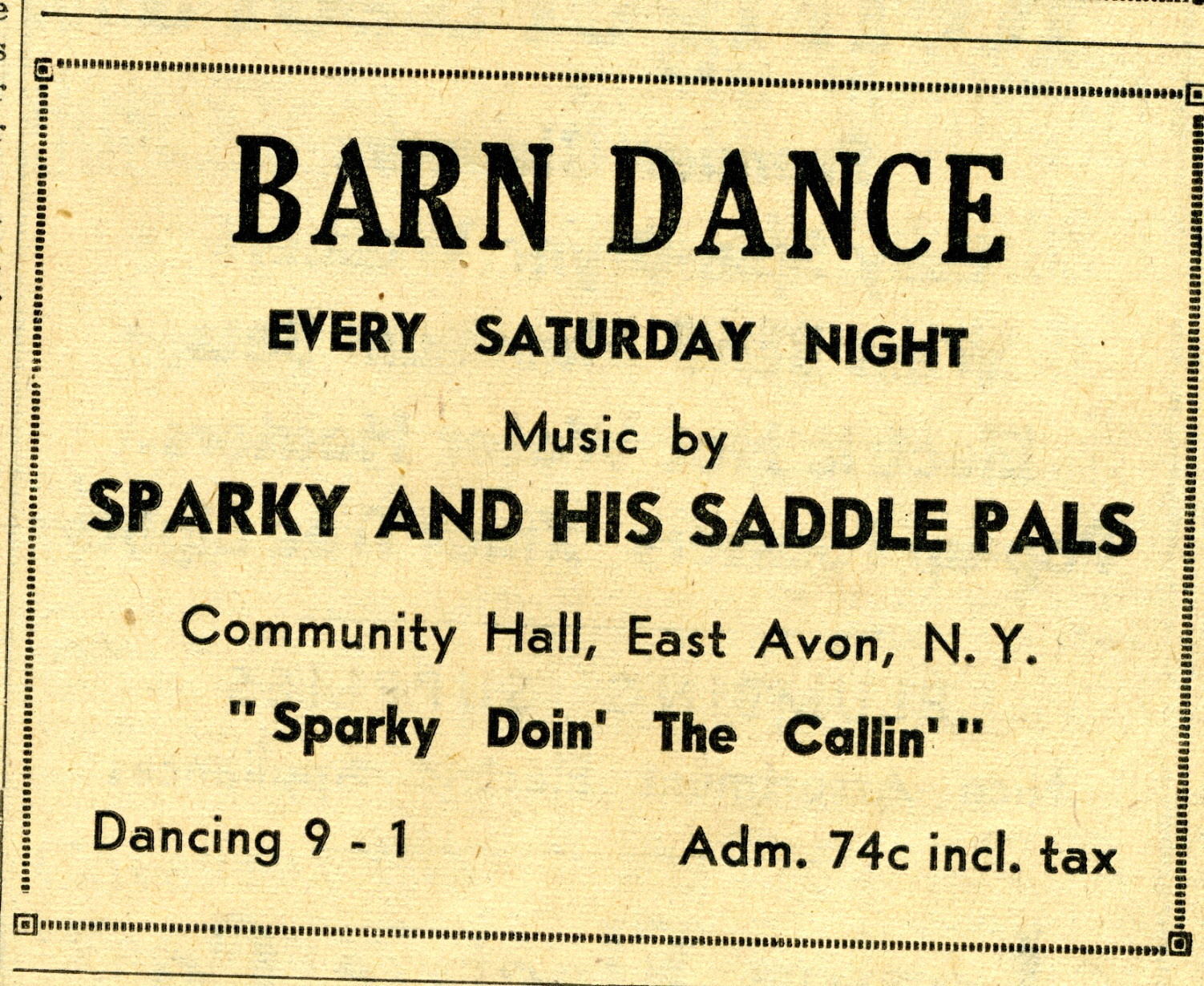A close-up photograph captures a nostalgic, slightly angled clipping of an old advertisement, likely from a newspaper or magazine, now yellowed with age. Encased within a dotted line border and additional black outer lines separating it from other ads, the ad reads in bold black text: "Barn Dance, Every Saturday Night, Music by Sparky and His Saddle Pals, Community Hall, East Avon, New York." In quotes, it highlights, "Sparky doing the calling." Further details note "Dancing 9-to-1" in the lower left corner and "Admission 74¢, includes tax" in the lower right. The ad’s intricate details and its well-preserved wording despite its vintage condition evoke a sense of historical charm.